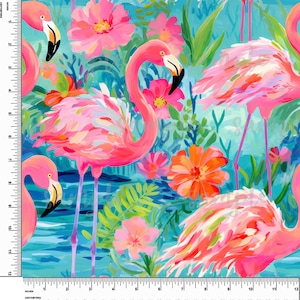This image is a detailed, square-shaped, 12-inch by 12-inch painting of flamingos in a slightly abstract style, marked with white rulers along the bottom and left sides, featuring black text and numeric markings. The painting features around five pink flamingos, some fully visible while others are partially shown, standing in shallow, aqua-colored water and surrounded by vibrant green plants, pink and red flowers, and blue and green grasses. The flamingos have white to orange beaks with black tips and display a mix of feather colors. The background includes fern-like foliage and a blue sky, evoking a scene reminiscent of Florida. Despite its vibrant and intricate details, the overall appearance of the painting is soft and somewhat blurry, enhancing its artistic charm.